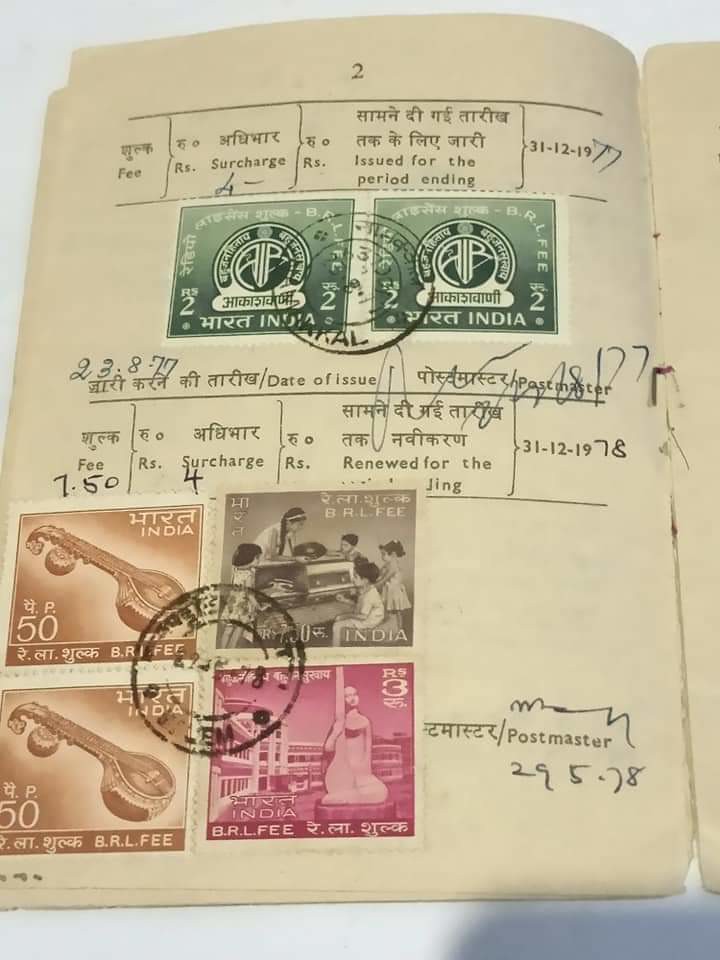This detailed photograph features a single object, predominantly occupying the frame, depicted against a white or off-white background. The object is an open page from a book, specifically the left-hand side. The page, which appears tattered and frail, showcases a blend of writings in a foreign language, likely Hindi, alongside English text. Key English phrases visible include "fee," "surcharge," "issued for the period ending," and specific dates such as "31-12-19" and "1978." The page is densely covered with various stamps: green circular stamps at the top, and a collection of stamps at the bottom in shades of brown, pink, and black. These stamps feature images such as native instruments, groups of children, and statues, implying an Indian origin. Hence, the document appears to be a postal or official ledger, meticulously documenting fees and dates, enhanced with stamps that indicate formal validation or postal processing.